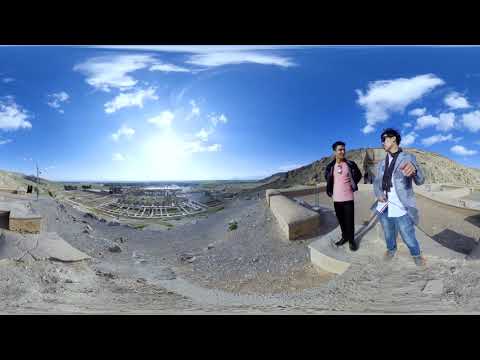In this outdoor image taken on a beautiful, partly cloudy day, two men are standing side by side on a rugged, high-elevation landscape that appears to be reminiscent of the Midwest, possibly New Mexico. The ground beneath them is mainly composed of sand and gravel, with rocks scattered throughout. On the right, a man with brown hair is wearing a blue jean jacket, blue jeans, and sunglasses, giving off a rugged, casual vibe. Next to him, another man is dressed in a dark-colored jacket, a pink t-shirt, and dark pants, adding a pop of color to the scene. The background features a high vantage point overlooking a large low building, and the terrain curves up into a hill on both the left and right sides. The sky is a perfect blue with a few scattered white clouds, completing the picturesque view. The two men, who exude camaraderie, could be friends or colleagues, possibly on an adventurous excursion to explore or document the area, which tantalizingly hints at being a historical or archaeological site.